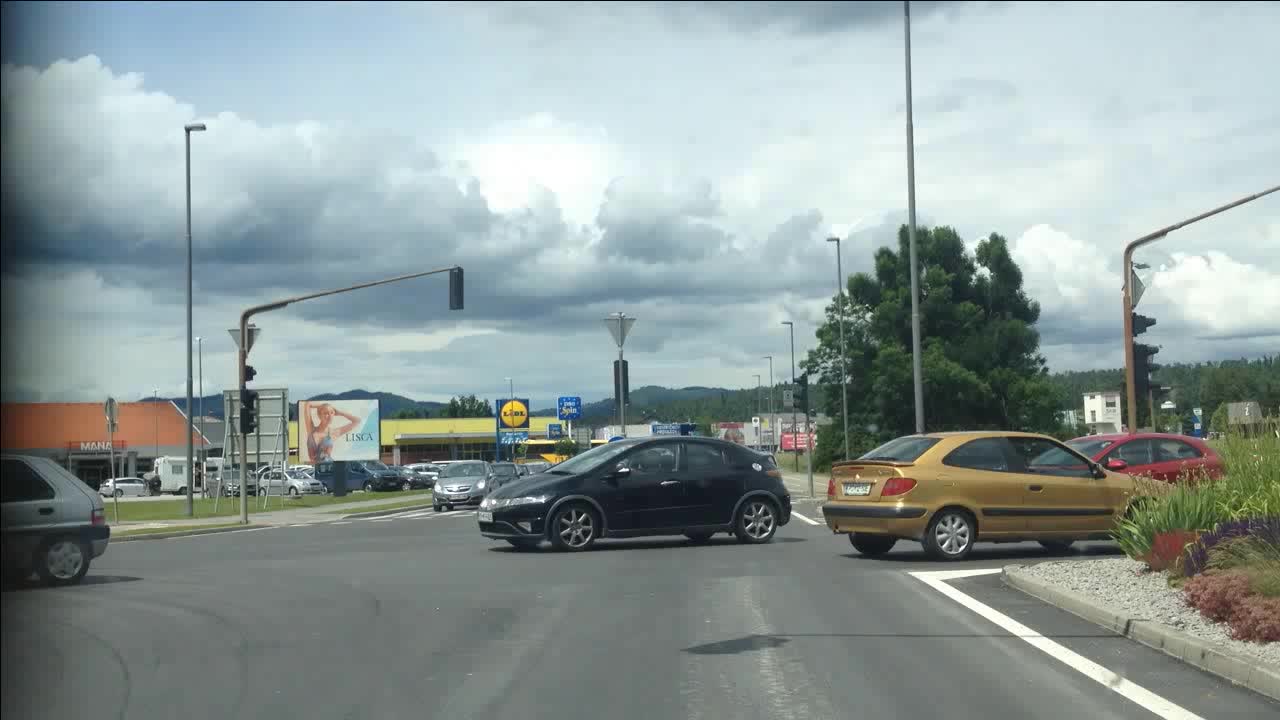A detailed street view photograph capturing an intersection in what seems to be a business or shopping district of a small town or city. The image is taken from a street facing an intersection where four cars are crossing perpendicular to the viewer's street, suggesting they have the right of way. Three of these vehicles are moving in one direction while the fourth heads in the opposite direction. In the distance, cars wait patiently for their signal to proceed. On either side of the street, small buildings line the area, though their specific purposes are indistinguishable. Trees are visible to the right, adding greenery to an otherwise commercial scene. Above, the sky is densely clouded, featuring a mix of blank gray clouds and more textured, white and dark gray fluffy clouds closer to the photographer, casting a subdued light over the image.